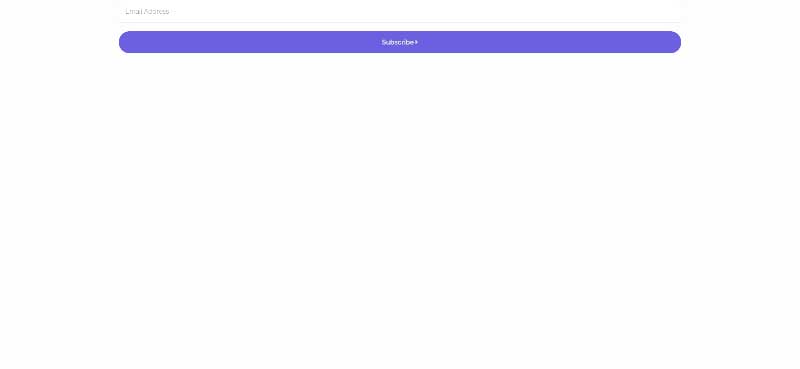The image features a clean, minimalist design on a white background. At the very top of the image, there is a light grey horizontal line that spans almost the entire width of the image. Directly below this line, in grey font, are the words "Email Address." Beneath the text, there is a prominent, wide purple button with the word "Subscribe" written in white capital letters. The button extends nearly from the left to the right edge of the image, aligning with the grey line above it. The remaining space below the button is an expansive white area, blending seamlessly with the overall background of the image. The color palette used consists primarily of grey, white, and a striking purple for the button.